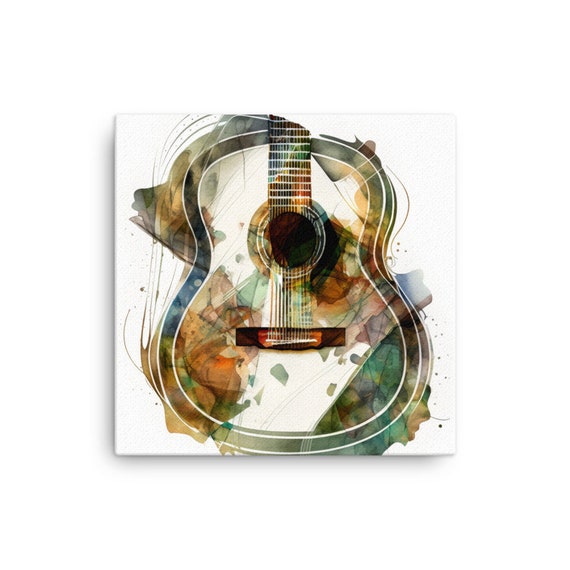The image depicts a highly stylized, top-down view of the body of an acoustic guitar. It occupies the center of a square, white canvas panel and is rendered with dynamic watercolor strokes. The guitar is delineated by a distinct white outline, with splashes and washes of vibrant and earthy colors including deep greens, various shades of brown, grays, oranges, and blues. These colors interlace and extend slightly beyond the guitar's silhouette, creating a sense of movement and depth. The main body features a translucent area, adding to the layered, watercolor effect. Visible within the body are white wire strings and the sound hole, while the neck, partially seen at the top, shares the same vivid color scheme. The overall aesthetic is that of modern wall art, blending abstract and realistic elements to convey both the form and essence of the guitar. The background remains a minimalist white, emphasizing the colorful complexity of the guitar itself.